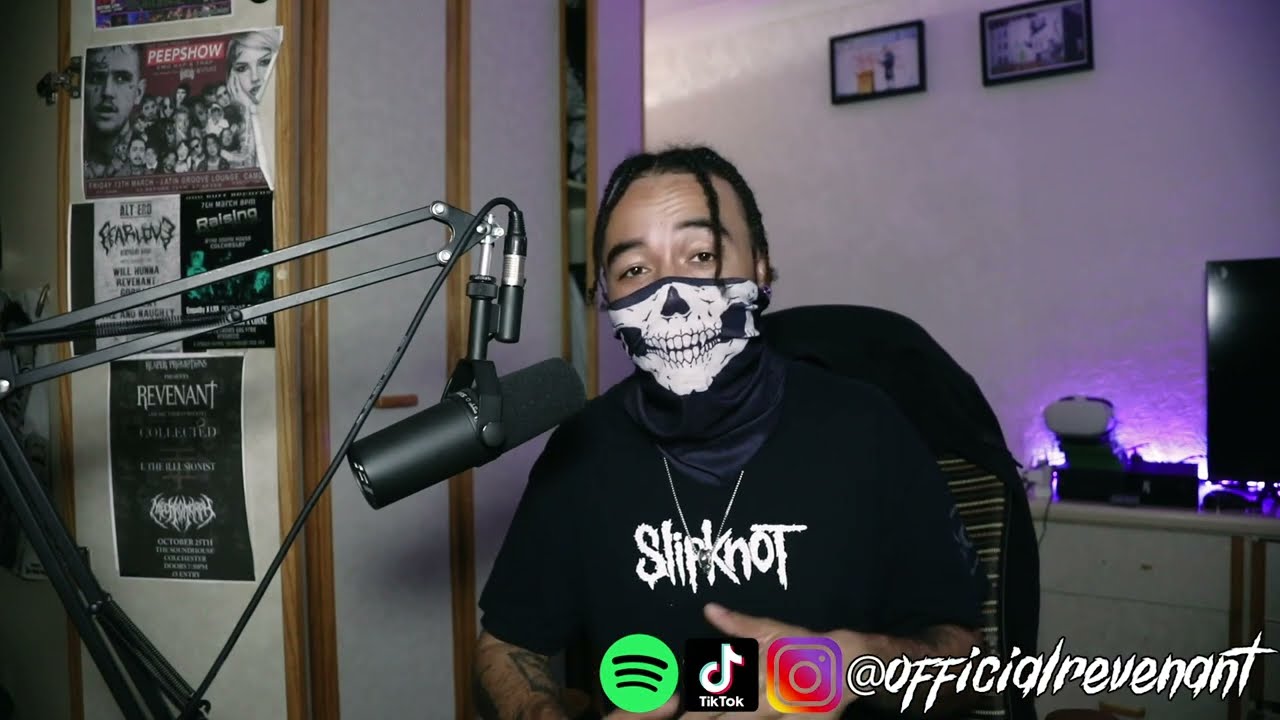In the image, a masked individual wearing a black and white Slipknot t-shirt sits at the center, engaging directly with the camera. The mask features a distinctive black rim and a white skull design with etched teeth. The person also has a few dreadlocks, with two hanging down the sides of their face. Positioned in a likely bedroom setting, the room includes various elements: a black microphone on a stand positioned to the individual’s left, posters and framed pictures adorning the brown and white wall to the right, and an entertainment stand in the background that holds a TV, an Xbox, and a VR headset illuminated by a purple light. Below the individual, the image prominently displays social media logos for TikTok, Spotify, and Instagram, each in their signature colors. The text "@official Revenant" is also visible, suggesting this might be an advertisement for their social media channel.